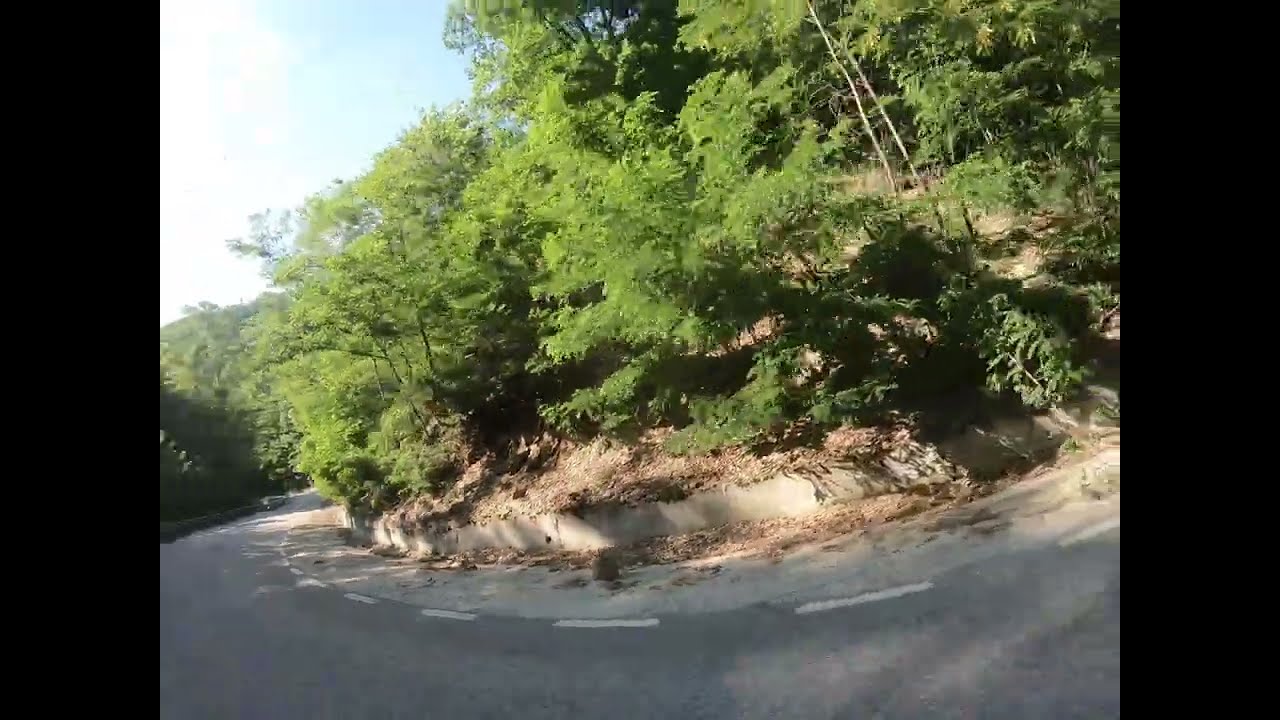This horizontally aligned rectangular photo captures an outdoor scene around a curved road. In the upper left corner, a partially blue sky filled with white clouds sets the backdrop. The middle and upper right part of the image features a dirt or mulch-covered, elevated median topped with a dense array of lush, green trees. The lighting is bright, casting dappled shadows from the trees onto the road below. The road, featuring white dashed lines between its two lanes, curves across the bottom right towards the left. There's potentially a larger vehicle, like a bus or truck, visible in the distant left. Flanking the sides of the picture are two thick black vertical borders, framing the scene. The road lacks shoulders, but a bike lane is striped off to the far right.